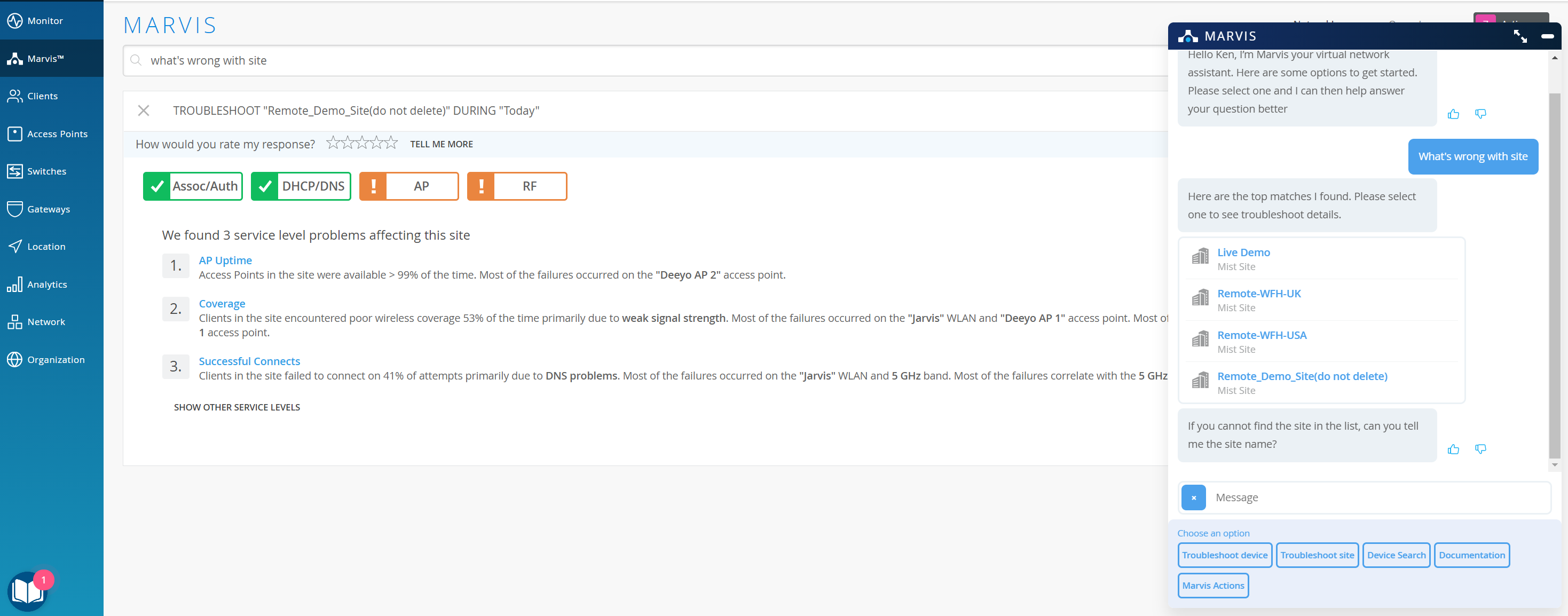The image depicts a detailed interface of the Marvis network management system. In the top left corner, "Marvis" is prominently displayed, with a blue navigation bar beneath it. The sidebar on the left categorizes various sections including Monitor, Clients (represented by two silhouettes), Access Points, Switches, Gateways, Location, Analytics, Network, and Organization. At the very bottom left, there is an icon depicting a white book within a red circle.

The main screen has a gray background and features a search bar at the top, complete with a magnifying glass icon and text that reads, "What's wrong with site." Below this, there are several options: "X," "Troubleshoot," "Remote," "Demo Site," and "Do Not Delete." Additionally, the interface includes a feedback section that prompts, "How would you rate my response," accompanied by five hollow stars labeled "One, Two, Three, Four," and a dollar sign beside "One."

Highlighted in green, a section labeled "Server/Auth" states, "GHCP is such a nice." Nearby, orange text labeled "EP" and another label "ARA" are also visible. A notification indicates, "We found three server-level problems affecting this site," with detailed insights including:

1. **AP Uptime:** Access points in the site were available more than 99% of the time, but most failures occurred on the DO AP2 access point.
   
2. **Coverage:** Clients experienced poor wireless coverage 53% of the time due to weak signal strength, with most issues originating from the drivers, WLAN, and DO AP1 access point.

This entire segment appears within a chat screen labeled "Marvis Chat."